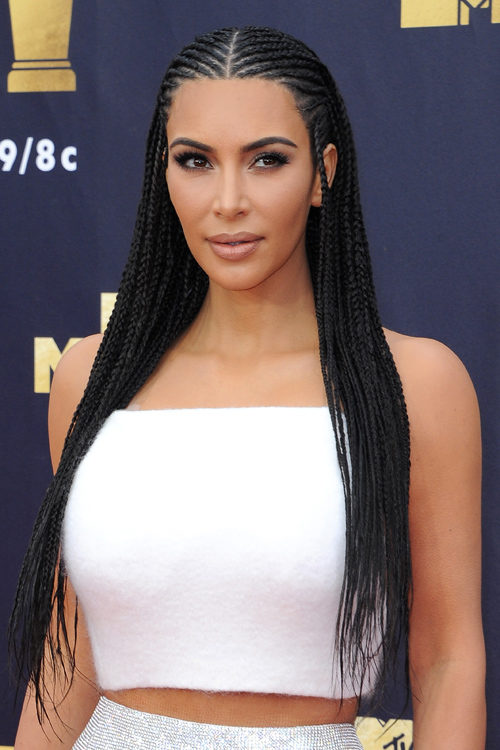In this photograph, Kim Kardashian is seen standing in front of a navy blue backdrop, suggesting she is attending a celebrity event, possibly an MTV award show. She is dressed in a strapless, fuzzy white halter top that exposes part of her midriff, and sparkling gray-white pants. Her hair is styled in thin cornrows that extend down to her waist. She looks directly at the camera with her thick brown eyebrows framing her brown eyes. The navy blue backdrop behind her features partially visible text reading "9/8C" and what appears to be the MTV logo, reinforcing the event's significance. The photograph captures her from the waist up, emphasizing her detailed and stylish attire and accessories.